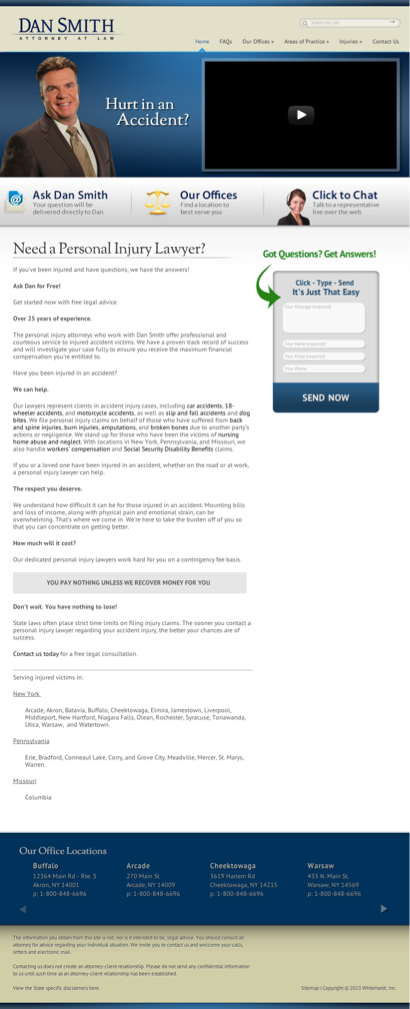Screenshot of a website showcasing the services of attorney Dan Smith, a personal injury lawyer. The top section features the heading "Hurt in an Accident?" next to a professional photograph of Dan Smith, who is dressed in a brown suit paired with a light brown tie. To his right, there is a video window with a play button; however, the video content is currently not displayed, leaving the screen black.

Below this, the site navigation includes three main sections: "Ask Dan Smith," "Our Offices," and "Click to Chat." Unfortunately, the accompanying text is too small to be legible. Further down, there's a descriptive section that addresses potential clients with the question, "Need a personal injury lawyer?" It reassures visitors that if they have been injured and have questions, Dan Smith offers free advice to help them get started. The text implies he has over 20 or possibly 35 years of experience in representing personal injury claims.

Highlighted within a gray box is the promise, "You pay nothing unless we recover money for you." This reinforces the notion that potential clients have no financial risk in seeking consultation. The site urges visitors not to delay and to take advantage of the free legal consultation offered. Dan Smith's attorney services cater to injured victims in New York, Pennsylvania, and Missouri. Overall, the website emphasizes reliability, respect, and expertise for those seeking legal assistance after an injury.